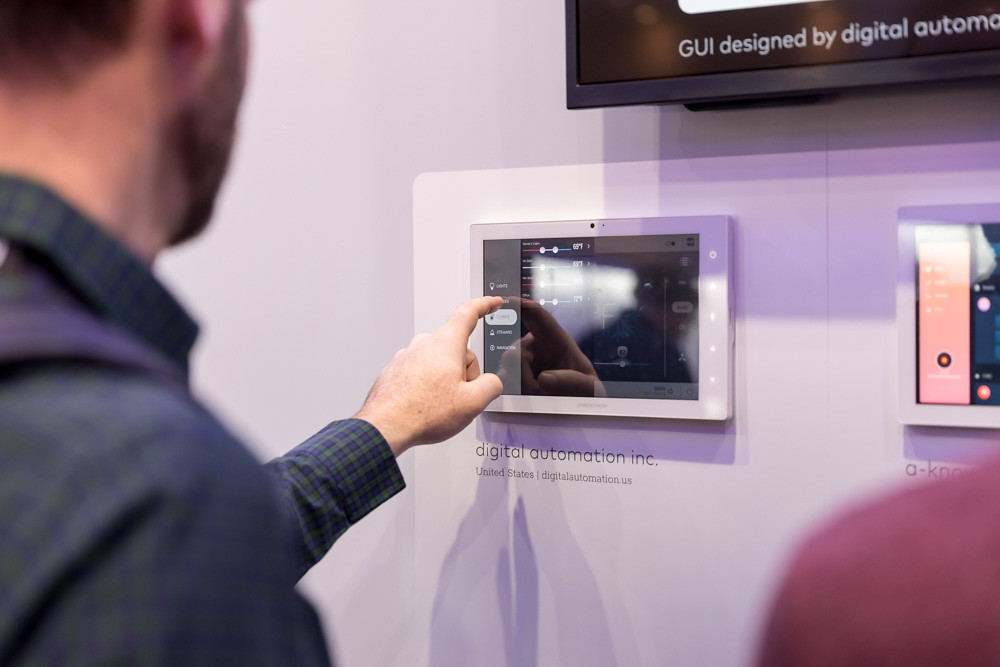The photograph captures an indoor scene featuring a white man with short brown hair and a light beard, wearing a dark green and blue plaid button-up shirt. He is situated on the left side of the image, with his head and shoulder visible, and his arm outstretched to interact with a touchscreen device mounted horizontally on a wall. The touchscreen, situated at the center of the image, has a dark interface with various gauges, sliders, and buttons, and a noticeable reflective glare. Below this central touchscreen, the text "Digital Automation Inc." is visible, followed by "United States Digital Automation dot US" in smaller black lettering.

To the right of this central device, there is another similar touchscreen, partially cropped out of the frame. Near the bottom right of the image, the shoulder of another person, wearing a red shirt, is barely visible and blurred. At the top right corner, a mounted black television screen is visible with the text "GUI Designed by Digital Automation" in white, although part of the screen is cropped out. The wall behind the devices and people is a mix of white and light brown or light gray tones, with shadows cast by the man and the mounted television.